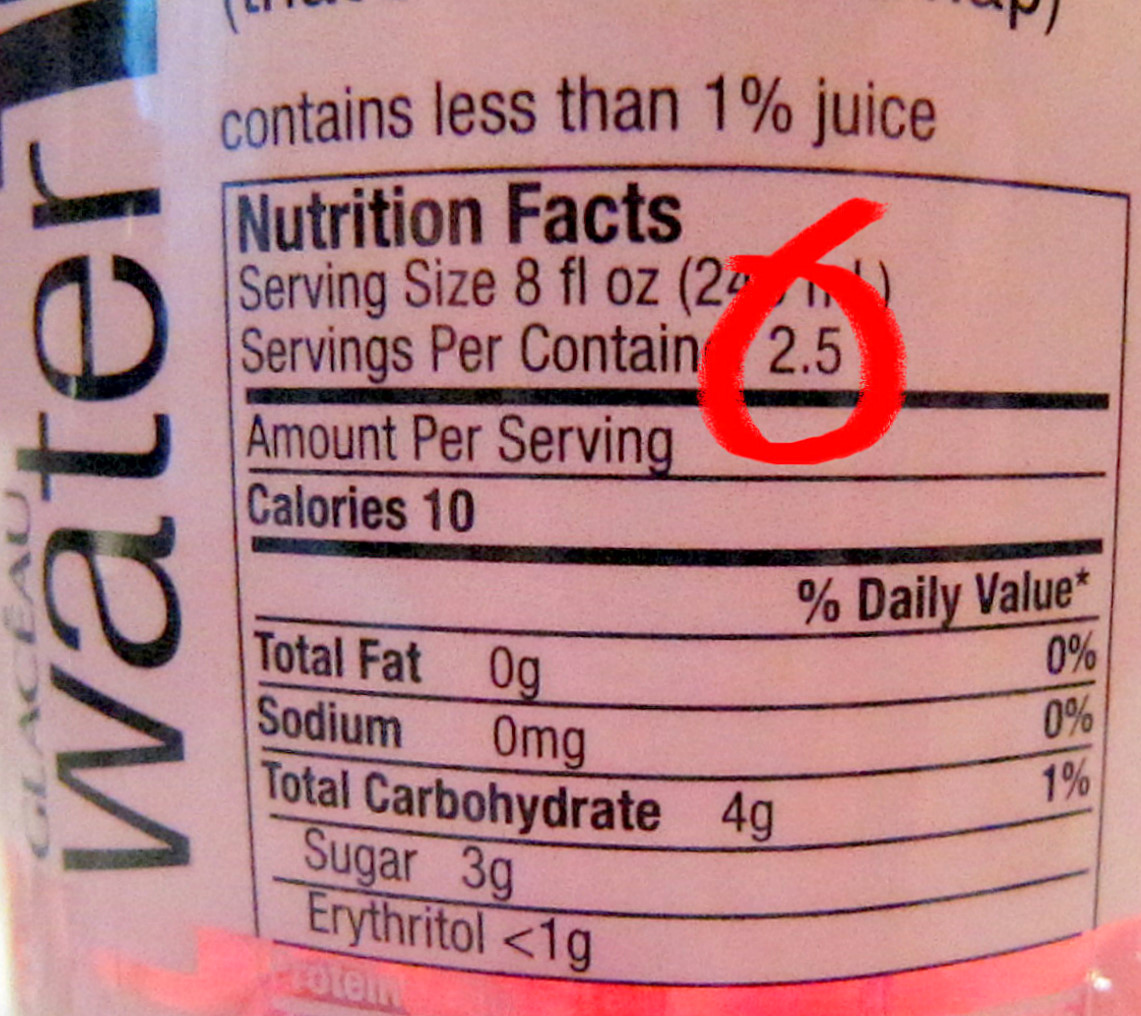This image depicts a beverage container label with a portion of the nutritional information highlighted. A circle is drawn around the "Servings Per Container" detail, which indicates there are 2.5 servings in the bottle. The beverage appears to be a fruit-flavored water, as it contains less than 1% juice and has added sugar. Each serving size is listed as 8 fluid ounces. Despite its presentation as a water drink, the label reveals it contains 10 calories per serving. The user's confusion is noted over the serving size and the practicality of drinking a partial serving.